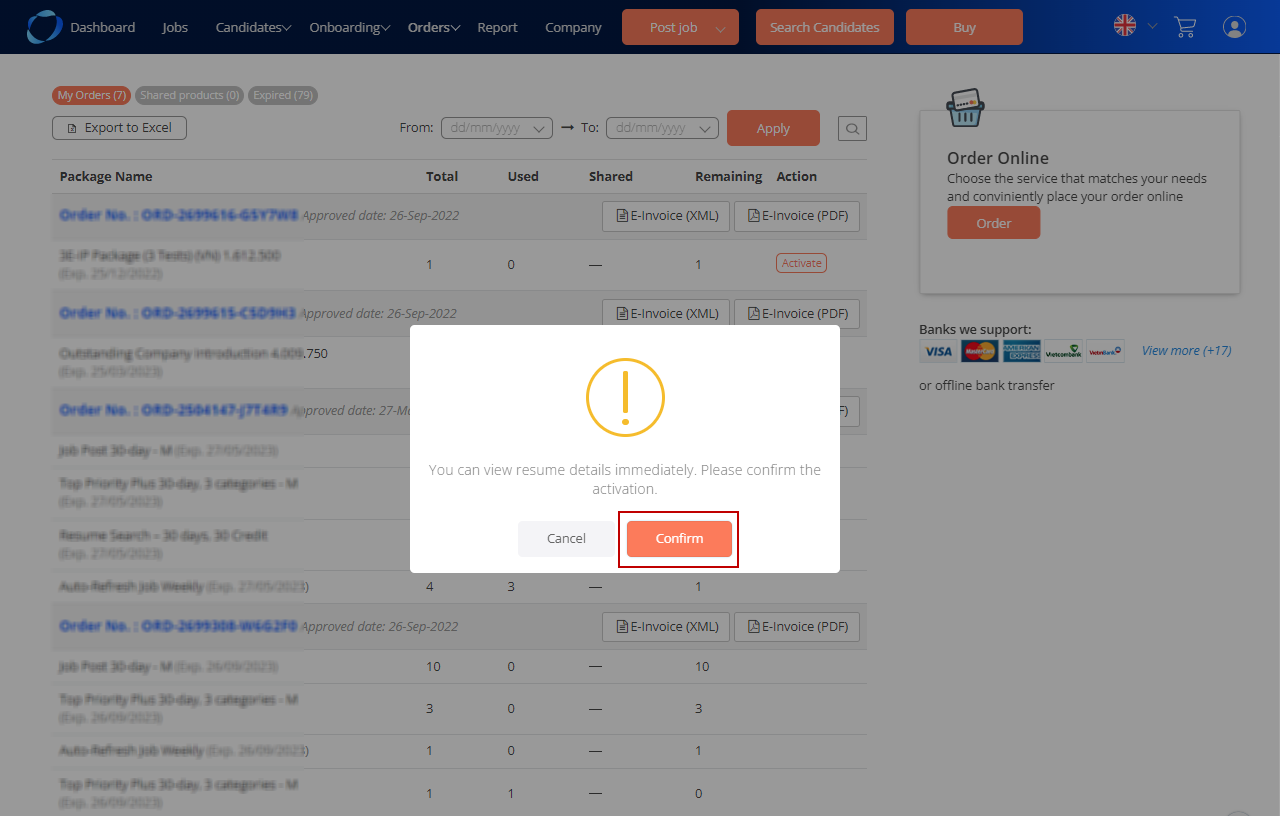Screenshot of a detailed dashboard interface:

At the top of the dashboard, a blue bar displays navigation options labeled as Dashboard, Jobs, Candidates, Onboarding, Orders, Reporting, and Company. Below this bar, three prominent orange buttons offer quick actions: "Post Job," "Search Candidates," and "Buy."

On the right side of the blue bar, there are several icons: a circular icon featuring the UK flag, a shopping cart, and a user icon. Beneath these, a white box provides information, stating "Order Online: Choose a service that matches your needs and conveniently place your order online," accompanied by a button to place an order.

The "Banks You Support" section lists supported payment options, including Visa, MasterCard, American Express, along with more options and a mention of 17 offline bank transfer methods.

At the top of the main page, an orange button labeled "My Order" indicates a count of seven. Nearby, a gray button labeled "Shared Products" shows a count of zero, and another gray button labeled "Expired" shows a count of seventy-nine. A rectangular button labeled "Export to Excel" and several date input fields are followed by an orange "Apply" button.

Central to the image, a white pop-up box with a golden exclamation mark inside a golden circle advises, "You can resume details immediately. Please confirm the activation." A red button at the bottom of the pop-up prompts users to "Confirm."